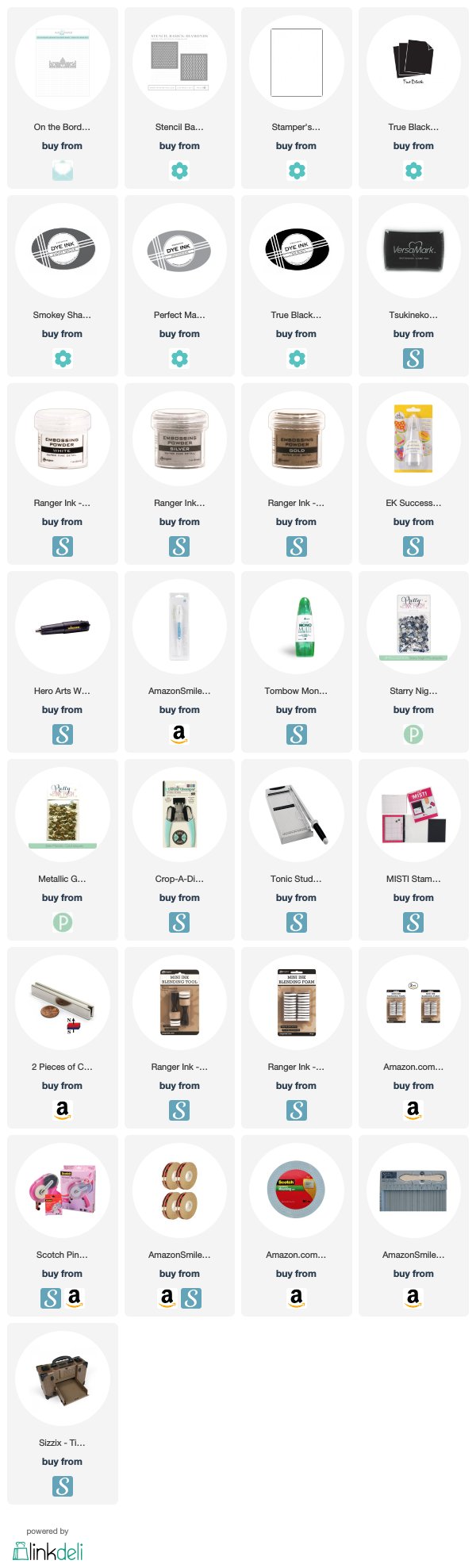The image appears to be a collage of multiple smaller images organized in at least four distinct rows. Each of these smaller images seems to depict various products, although the specifics are difficult to discern due to their small and hazy nature. Most of the images have a small emblem at the bottom, resembling a blue star, and some feature icons resembling an "A," potentially indicating an Amazon product, or a blue square with a white "S." Among the indistinct images, there seem to be containers, note cards, and possibly tape, suggesting that the products might be office supplies or similar items. The text accompanying these images is very small and hard to read, further contributing to the overall challenge in identifying the exact nature of the depicted items.